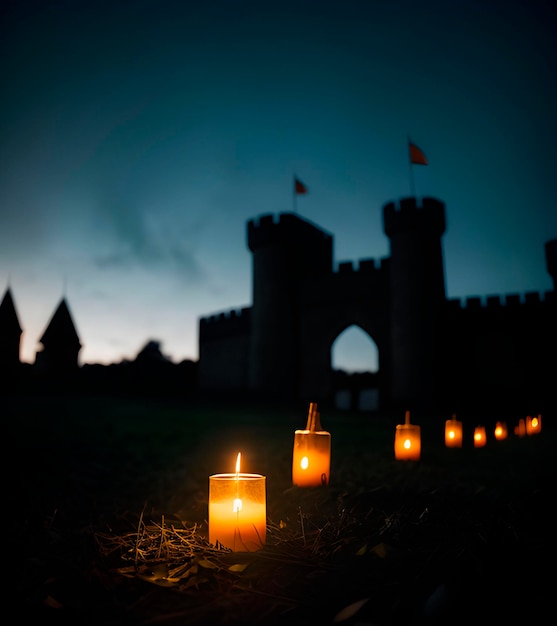Against a twilight sky that transitions from white on the horizon to deep blue and black overhead, an ethereal scene unfolds. The ground is covered in a brushy mix of twigs and dead vegetation, and set upon it are seven or eight lit candles, each housed in glass jars and topped with what appears to be a cinnamon stick. The predominant colors of the image include varying shades of blue, black, white, orange, brown, and flecks of green. In the background, the silhouette of a grand castle with distinct architectural elements, including two tall, cone-shaped turrets and several flag-topped structures, stands tall and mysterious against the fading light. The fortress-like walls, adorned with rectangular and round towers, add to the scene’s medieval ambiance. The sky suggests an early evening setting, just after the sun has dipped below the horizon, casting a minimal yet evocative light over the landscape. There are no people, animals, or vehicles present in this tranquil, picturesque scene.